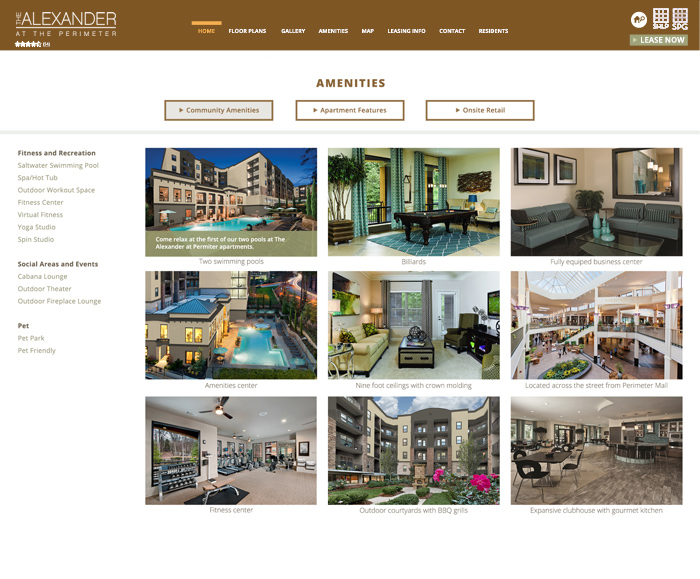This screenshot from a website showcases the amenities offered by "The Alexander at the Perimeter." The website's navigation bar at the top includes buttons for Home, Floor Plans, Gallery, Amenities, Map, Leasing Info, Contact, and Residence. A prominent "Lease Now" button is located near the upper right-hand corner. 

The central portion of the screenshot highlights the "Amenities" section, with the "Community Amenities" tab selected. Additional tabs for "Apartment Features" and "On-Site Retail" are also visible but not selected. Displayed below are labeled photos of nine featured amenities: two swimming pools, a billiards room, a fully equipped business center, an amenity center, nine-foot ceilings with crown molding, a location across the street from Perimeter Mall, a fitness center, outdoor courtyards with barbecue grills, and an expansive clubhouse with a gourmet kitchen.

On the left side of the screenshot, there are detailed descriptions covering various aspects such as fitness and recreation, social areas and events, and pet policies.